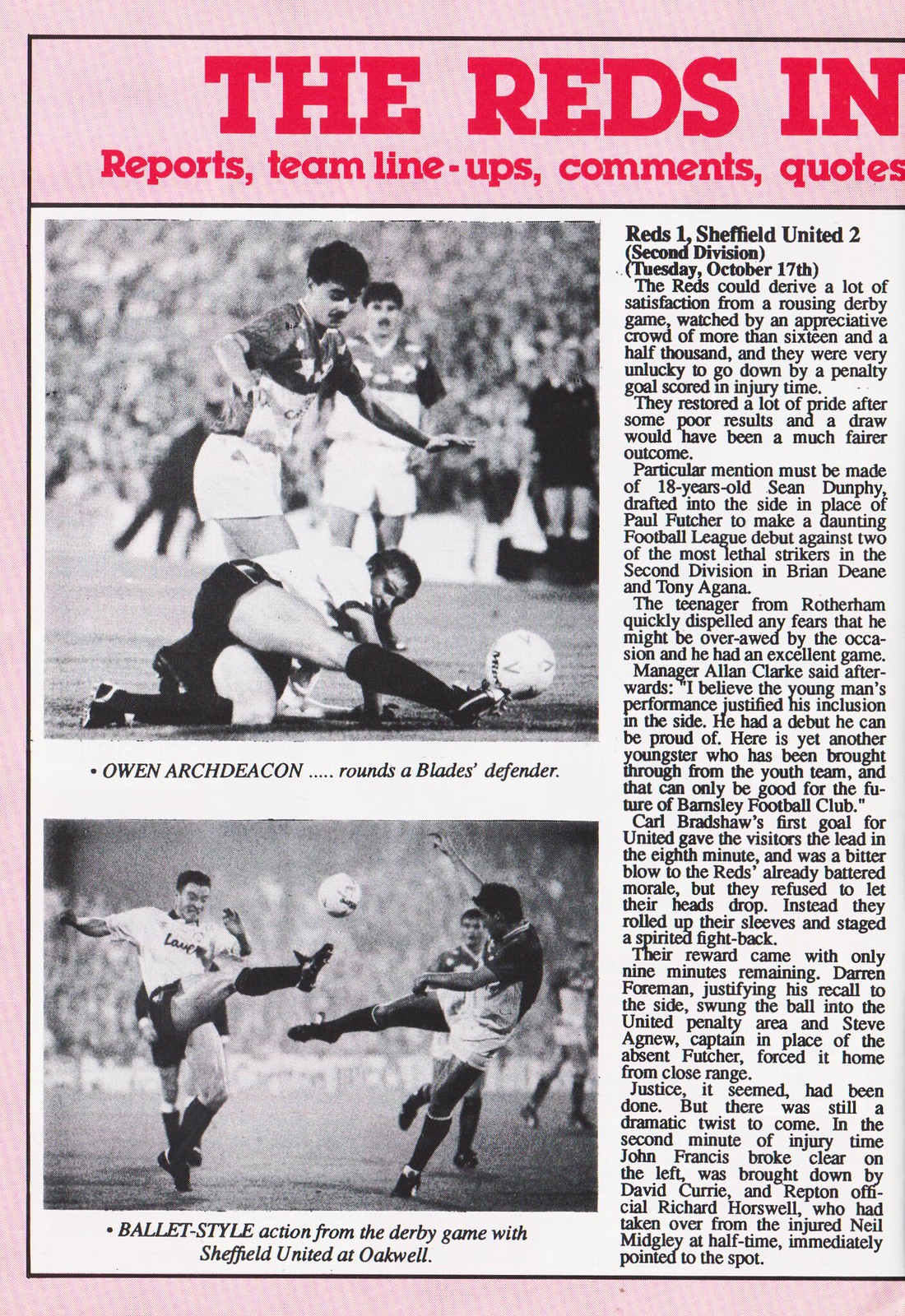The image is a newspaper clipping from an old English football magazine, primarily in black and white but bordered with pink. The header, set against the pink background and written in red block letters at the top, reads: "The Reds in reports, team lineups, comments, and quotes." Below this, the page features two black and white action photographs. In the top photo, a dramatic scene unfolds with three players: one player on the ground in a split, kicking the ball, while another player stands over him, and a third looks on. The bottom photo captures a player in white shorts performing a high kick, while an opponent attempts to block him. A caption under the photos notes, "Ballet action from the derby game with Sheffield United at Oakwell." To the right of the images, there's a news column in black text against a white background, completing this detailed chronicle of the soccer match.